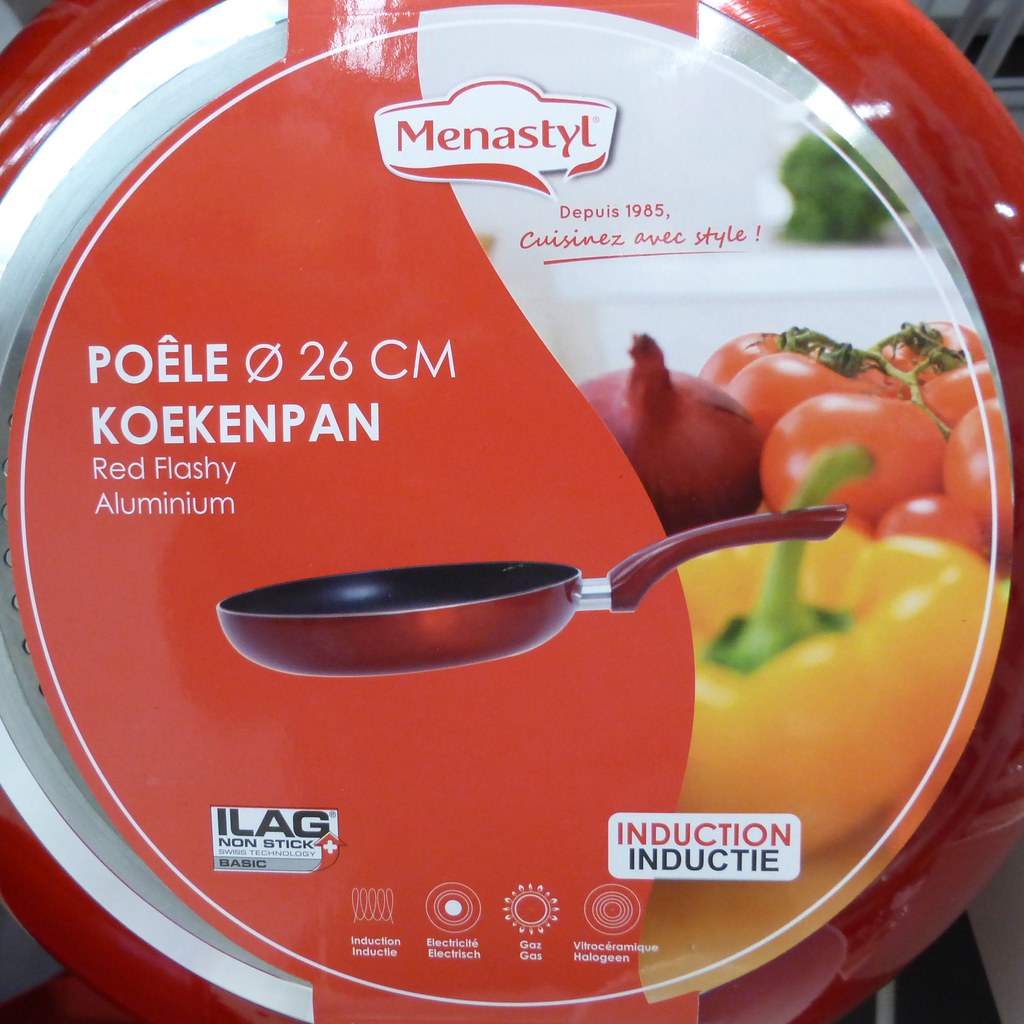A red frying pan is shown, viewed from its underside. The pan features a metallic center and a circular paper label taped to the bottom. The label has a red background and prominently displays the words "Red Flashy Aluminum." At the top of the label, there is a logo that reads "Menace Still." On the right side, the label showcases images of tomatoes, a red bell pepper, and a red onion. Above these images, the phrase "Cuisines Avec Style" is written, suggesting a stylish kitchen product. At the bottom right corner of the label, the words "Induction" and "Inductive," followed by "Electric, Gas, and Halogen" indicate the pan's compatibility with various heating methods.